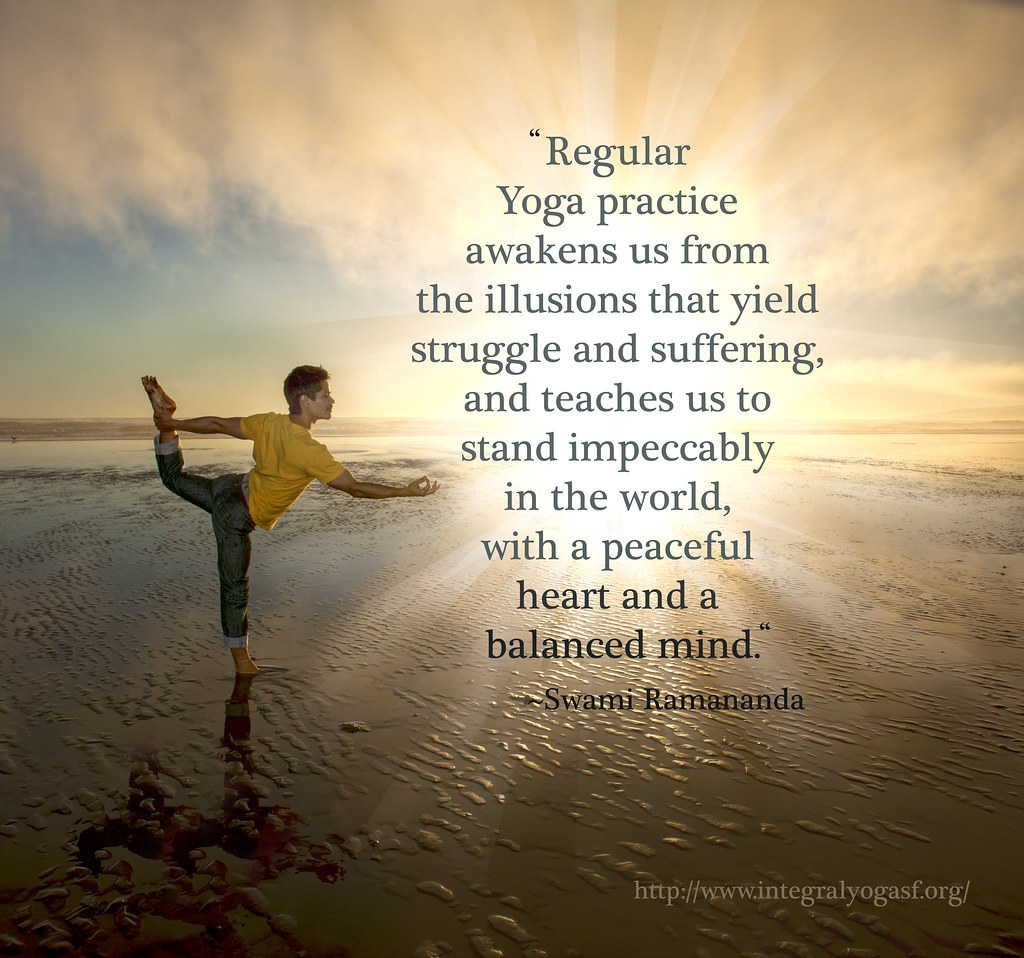In this full-color, professionally taken photograph used as a motivational poster, a man performs a yoga pose on a serene beach. He stands on one leg with his other leg bent backward, holding his ankle with his left hand. His right arm extends forward with his forefinger and thumb touching, creating a sense of balance and focus. The man is dressed in rolled-up blue jeans and a white t-shirt, standing ankle-deep in the wet sand as gentle waves lap the shore.

The backdrop features a spectrum of natural hues, including shades of brown, pink, peach, yellow, blue, and white, blending the sky and beach into a calming panorama. Centered next to the man is an inspirational quote by Swami Ramananda that reads, "Regular yoga practice awakens us from the illusion that yields struggle and suffering, and teaches us to stand impeccably in the world with a peaceful heart and a balanced mind." Below the quote is a website link: [http://www.integralyogaasf.org/](http://www.integralyogaasf.org/), suggesting it is an advertisement promoting the teachings of Integral Yoga.